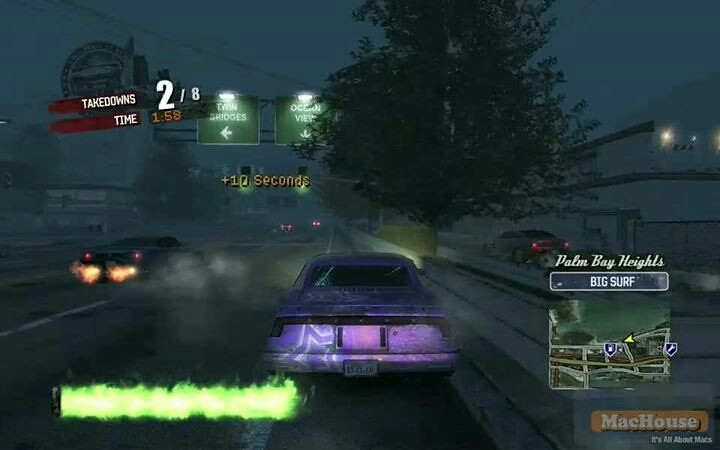This color image, likely a scene from a video game, depicts a dark, nighttime roadside setting. At the center of the image, we see the rear of a purple car. Just ahead and to the right of the car stands a dark tree, casting a shadow over the right side of the road. To the left side, the headlights of another dark car emit a yellow glow, providing a faint illumination. There seems to be another vehicle positioned to the right, slightly beyond the tree.

The road is flanked by buildings on both sides, though they are obscured by darkness, blending into the nearly black sky and road. In the upper left corner of the image, some road signs are visible. Among them are red signs displaying numbers and text: "time and taken 2 over 8, 1 over 1.5." Below these are green signs with white text and arrows pointing right and downward, accompanied by unreadable yellow print.

A faint, blurred green light or text appears in the bottom left-hand corner, while the bottom right-hand corner features a map, possibly indicating the car's location within the game. Adjacent to the map is a small orange logo with white text that reads "Machaus." The overall darkness of the scene makes many details challenging to decipher, contributing to the mysterious and immersive atmosphere typical of video game environments.